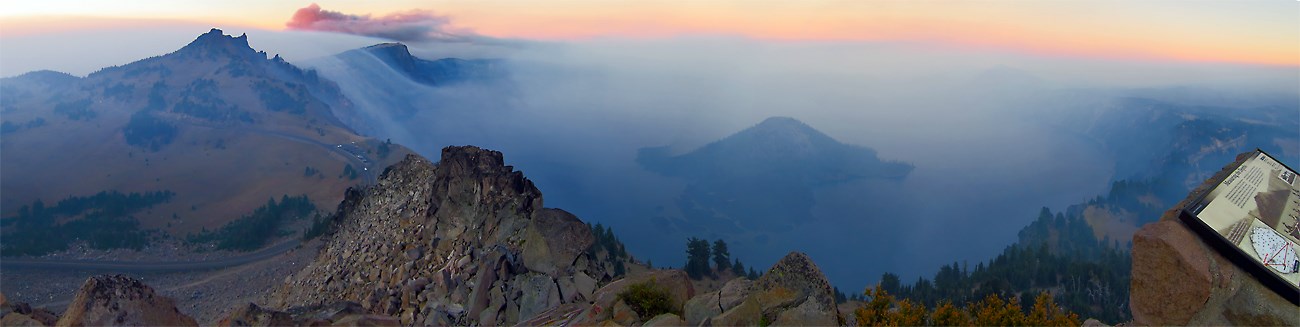A breathtaking mountain range scene captured during sunset, with an orange hue illuminating the horizon. The craggy, barren mountains, likely composed of shale or similar stone, are seen in the background with a placard on the right that probably details the ranges. The valley below is shrouded in mist and fog, enveloping some of the mountaintops and adding to the ethereal quality of the scene. A road winds its way through the left side of the crater-like formation, while a small hill peaks out from the fog inside the crater. Clouds hover above the mountains, adding depth to the sky. The overall scene is devoid of people, emphasizing the vast, deserted beauty and tranquility of the mountainous landscape.